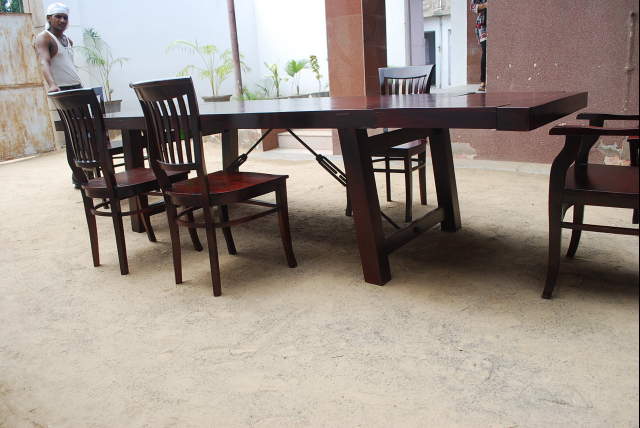In the image, there is a long, dark wooden dining table, stretching from left to right in the upper part of the photograph. The table has two thick wooden legs and appears to be very sturdy. Around the table, there are five chairs – two on the left-hand side, one at the back, and a partially visible chair on the right-hand side. The chairs are not perfectly aligned under the table, suggesting they’ve been recently used and not yet neatly arranged.

The table is situated either in an indoor room with large windows or in an open-air area, as there is natural light, greenery, and what seems to be another building with a door and a sign in the background. The floor in front of the table is a greyish-beige color with black speckles, potentially carpeted, though it's hard to tell for certain. The walls behind the table are a reddish-brown color, along with a large square column.

In the upper left corner of the image, there's a man standing next to the table. He appears to be wearing a sleeveless shirt and a white head covering, possibly a do-rag. He has dark skin, appears muscular, and his features suggest he might be Latino or Hispanic. To the top left, there is another wall texture, beige and white, along with a tiny green sign at the very uppermost corner.